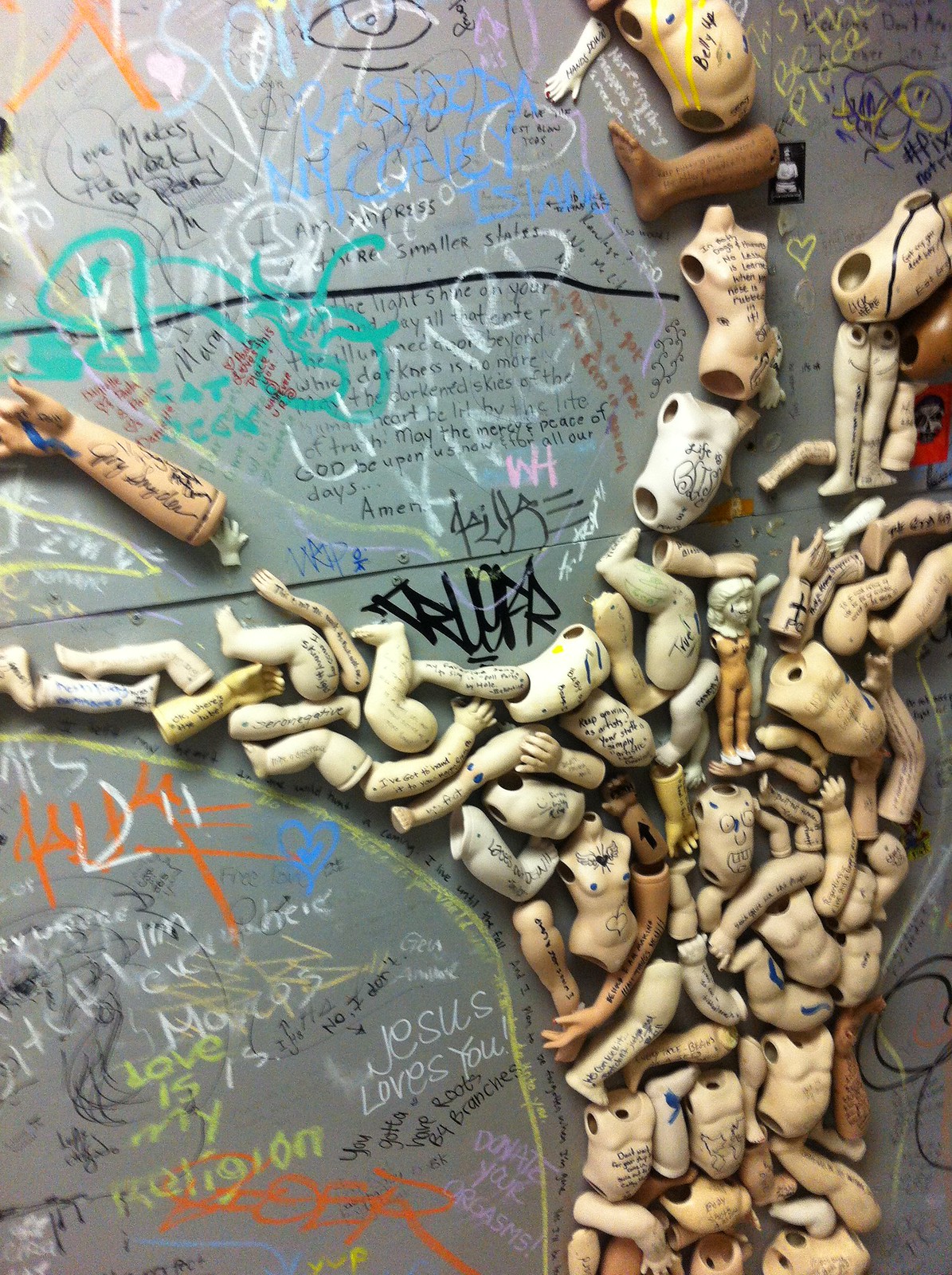This vertical, rectangular artwork is a detailed and abstract collage, primarily featuring a three-dimensional tree adeptly fashioned from an assortment of broken doll limbs and torsos. The tree, constructed from beige, gold, and brown doll parts, grows from the bottom right corner, with its main branch extending to the center left, another branch reaching the top right, and two smaller branches stretching straight up and towards the top left. Each of these limbs is inscribed with various sayings and drawings in black ink.

A pale yellow outline defines the tree trunk, and this line continues to the bottom left, which is also delineated with a yellow margin. The artwork's background is a dark gray cement board, heavily adorned with scattered graffiti and chalk writings. Notable phrases included in the collage are "Love is my religion," "Jesus loves you," "You gotta have roots before branches," and the eclectic "Donate your orgasms." The upper sections of the image, especially the top center between the branches, feature additional phrases like "Lizard King" and "White Chalk." The blending of the chalk graffiti with the doll parts creates an intricate pattern of modern and abstract artistic expression.